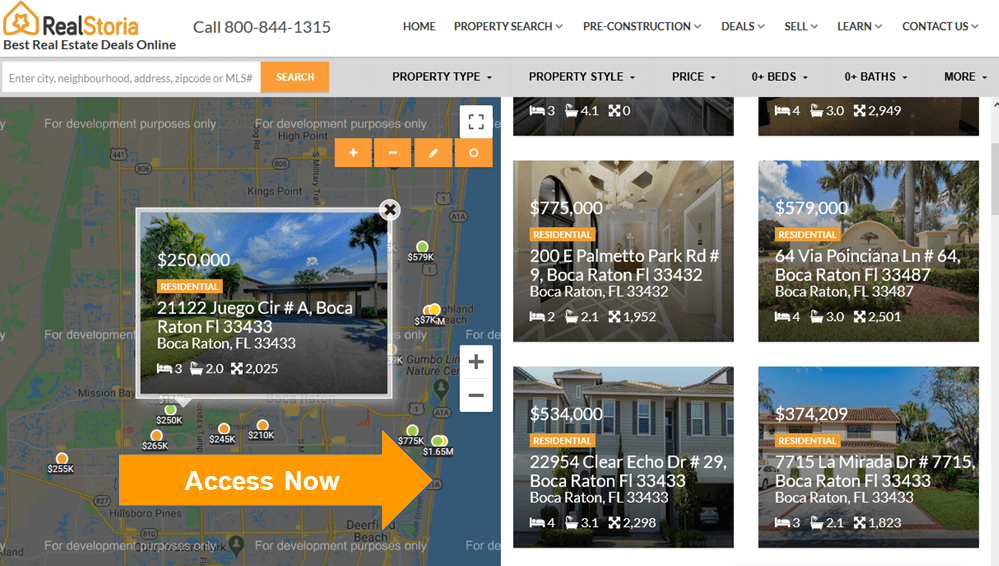The image appears to be a screenshot from a real estate website designed with a landscape orientation, approximately twice as wide as it is tall. In the upper left corner, the website features a distinct logo shaped like an upside-down heart or a guitar pick, wrapping around to form an outline of a star. The logo is mainly white with the outline and star rendered in an orange color.

Next to the logo, the website's name "Real Storia" is displayed in a bold font, with "Real" in black and "Storia" in orange. Both words are slightly compressed together, almost appearing as one. Below the name, a tagline reads "Best Real Estate Deals Online" in smaller, black text. To the right of this tagline, there is a contact number: "Call 800-844-1315". Further to the right, a navigation menu lists seven options: Home, Property Search, Reconstruction, Deals, Sell, Learn, and Contact Us.

The main section of the webpage is divided into two distinct areas. On the left side, there is an interactive map populated with approximately ten pins, each representing different real estate listings, identifiable by the price tags displayed below the pins. A prominent orange arrow with the text "Access Now" encourages users to click on one of the pins for more information.

On the right side, there is a grid showcasing four different property listings, providing users with a quick glance at available properties.